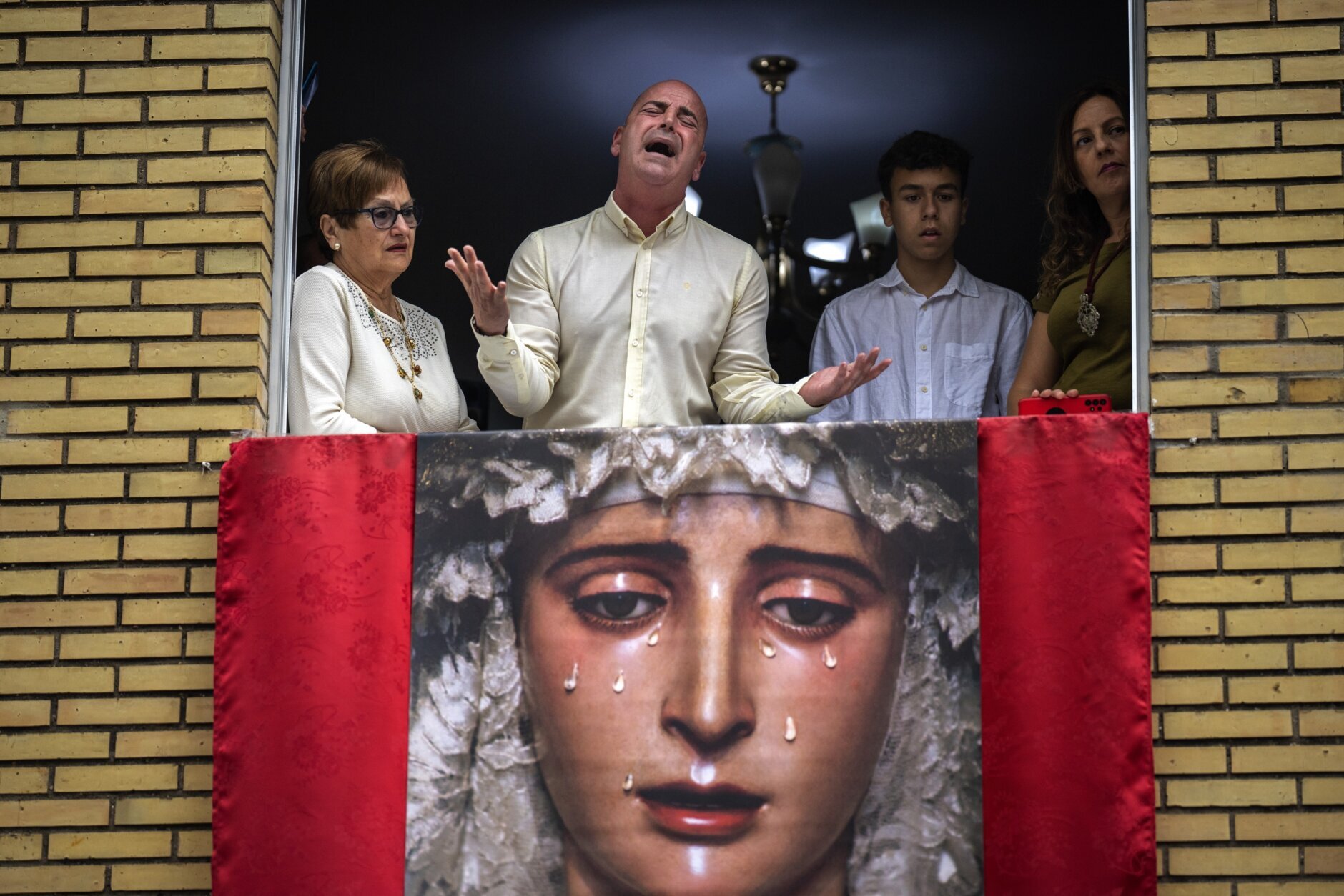The image depicts a poignant scene framed within the light brown brick walls of a building. Four people—a family consisting of an older woman, an older man in a yellow shirt with his arms stretched out dramatically, a younger man, and a younger woman in a red shirt—stand in an open window. They all have somber expressions, seemingly looking down at something on the street below. Behind them is a dark purple ceiling with a light fixture hanging down. Draped over the edge of the window is a striking art piece of a weeping woman. The woman's face is adorned with white feathers and bordered by bold red stripes. Her tears, resembling sparkling jewels or milk, flow down her cheeks. The woman has red lips, dark eyebrows, and dark eyes, and she wears a white scarf covering her head. This compelling blend of emotions suggests the family is experiencing a distressing or traumatic event.